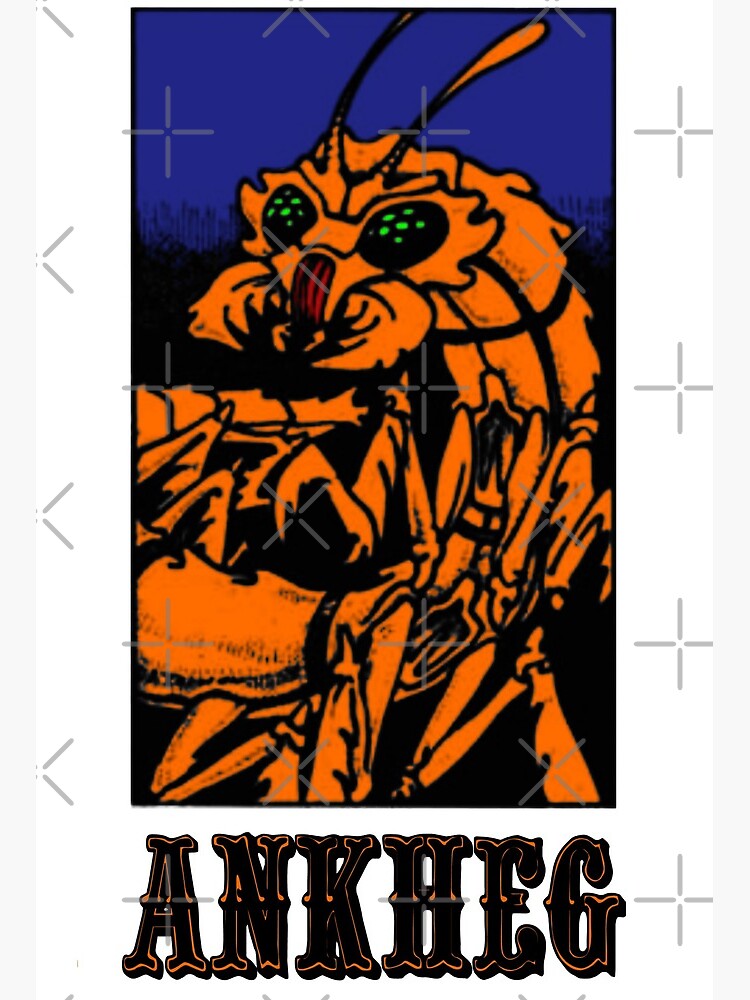This poster features a vertically aligned rectangular illustration of an orange insect identified as an "ANKHEG" at the bottom in bold, ornate black font edged with a thin orange outline. The image is bordered by a black frame, and the upper section of the background is filled with a dark blue, almost navy hue, while the area behind the insect remains pitch black. The insect, drawn in vibrant orange with intricate black outlines providing shading and detail, has prominent black eyes with tiny neon green dots, and a slightly red-tinted area around what appears to be its nose or tongue. Orange antennae extend back from its head. The insect's body is somewhat indistinguishable due to the dense black lines, and it appears to be curled with its face directed towards the viewer. Encasing the entire illustration is a white border, adorned with gray cross-shaped and x-shaped patterns that give a watermark-like effect, some of which extend into the main image. The light gray bars on the left and right sides contribute to this elaborate border, enhancing the overall presentation of this insect-themed artwork.